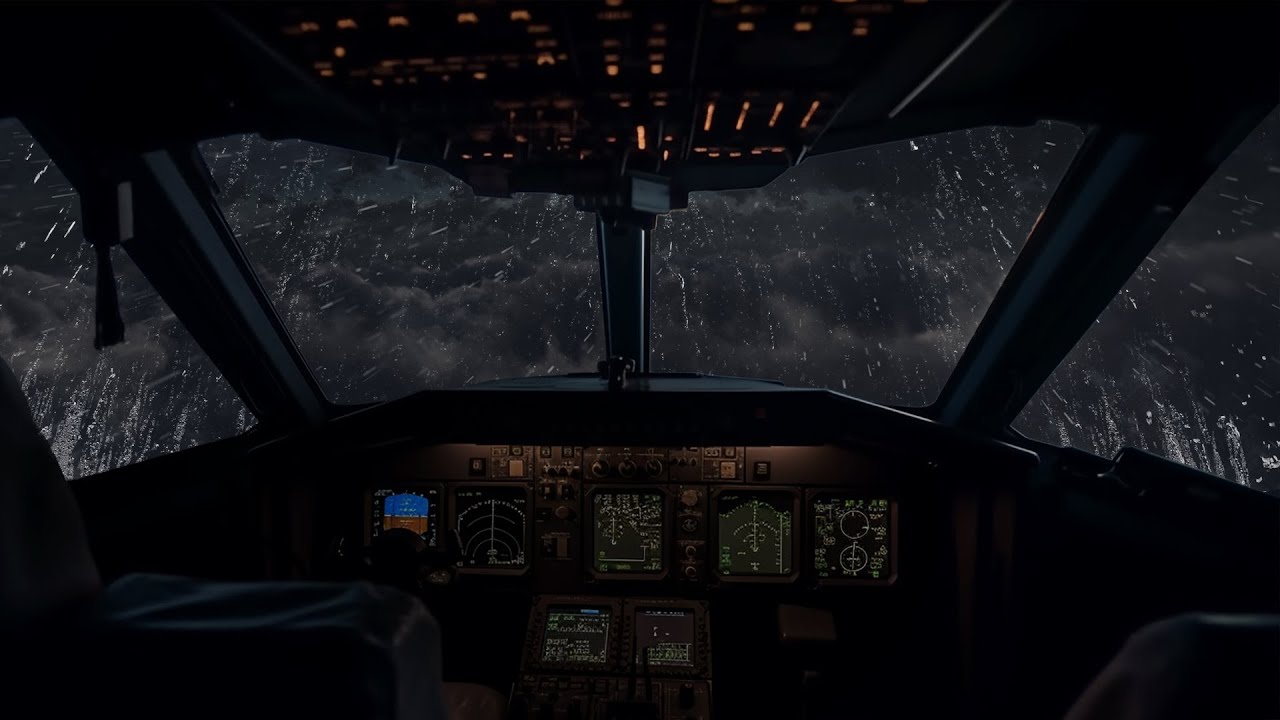The image depicts a dimly lit cockpit of an airplane during a stormy flight. Outside the multi-sectioned windows, heavy rain lashes against the glass, creating a very dark and menacing atmosphere with black and gray clouds looming in the sky. Inside the cockpit, there are no people visible. However, two empty black seats can be seen. The interior is illuminated by various control panels and screens, some displaying indistinct information. Numerous buttons, knobs, and lights are situated both on the dashboard and overhead, adding to the complex array of instruments used for flight navigation. The overall scene conveys a sense of tension and unease.